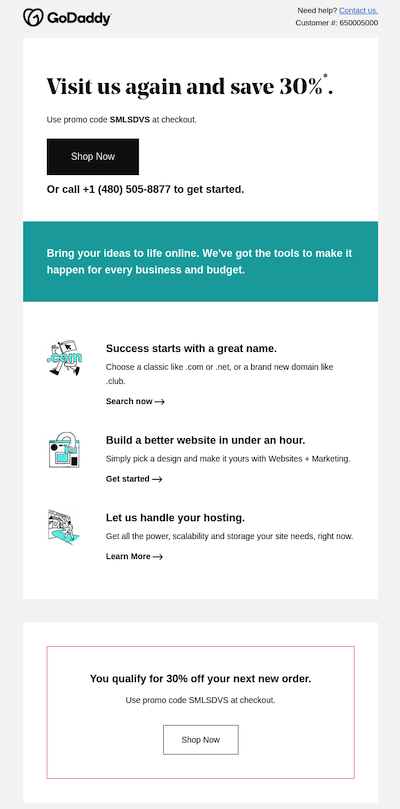The promotional image features a sleek, multi-colored design and includes a variety of marketing messages. At the top, the GoDaddy brand is prominently displayed alongside a "Need Help? Contact Us" prompt in blue. Below that, there's a customer number specific to Amazon, followed by a discount offer encouraging repeat visits with the text, "Visit Us Again and Save 30%, Use Promo Code SMLSDVS at Checkout," highlighted within a red rectangle.

In the center, a prominent black rectangle contains a "Shop Now" button in white, alongside contact information: "Or Call +1 (480) 505-8877 to get started." Adjacent to this, a vibrant teal rectangle bears the motivational caption, "Bring Your Ideas to Life Online. We've got the tools to make it happen for every business and budget."

Additional sections include:
- "Success Starts with a Great Name" with a "Search Now" prompt and right arrow,
- "Build a Better Website in Under an Hour," with a "Get Started" button and right arrow,
- "Let Us Handle Your Hosting," complemented by a "Learn More" button and right arrow.

The lower portion reiterates the discount offer, emphasizing, "You Qualify for 30% off Your Next New Order, Use Promo Code."

This well-organized, colorful layout aims to guide potential customers through various services offered by GoDaddy while providing incentives for engagement and purchase.